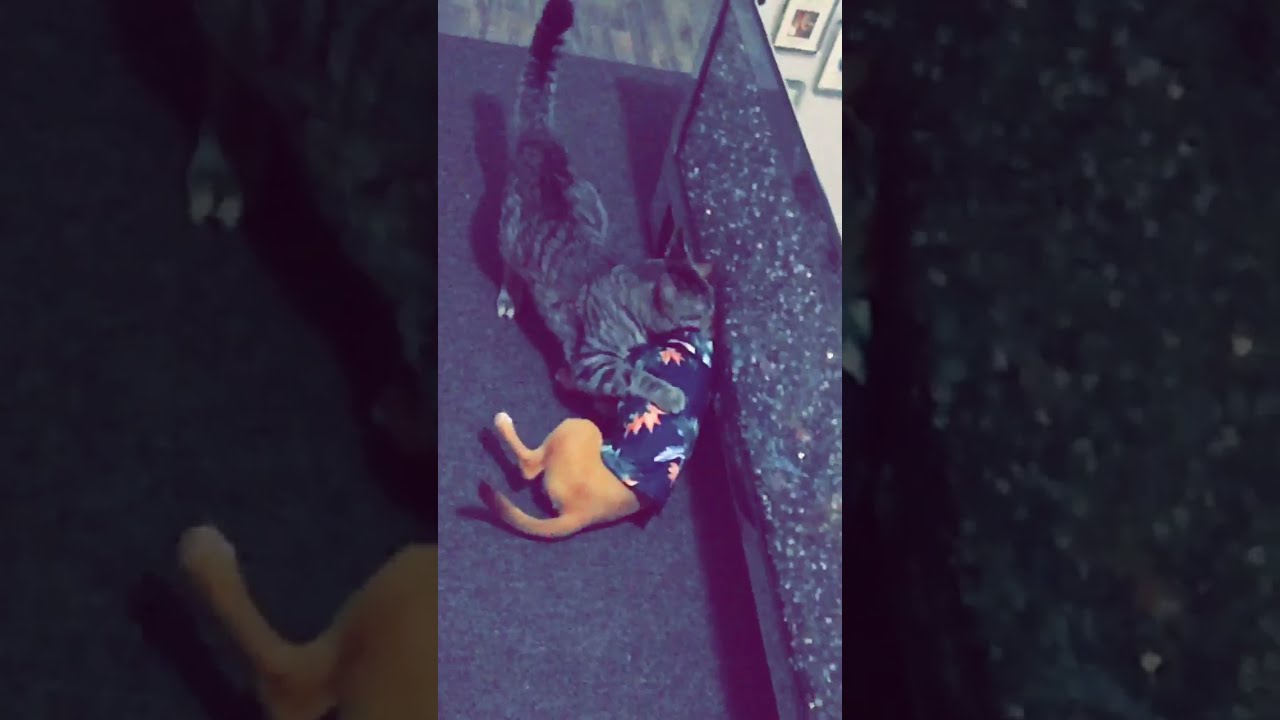In this vivid photograph, a large gray tabby cat is perched aggressively atop a small brown dog, the cat seemingly having the upper hand in what looks like either a play-fight or an intense tussle. The dog, whose face is obscured by the cat, lies on a gray floor, wearing a distinctive dark blue Hawaiian shirt adorned with pink flowers. The dog has light brown fur, white feet, and a long tail tipped in black. The scene appears to be set indoors, beside a cabinet. The image is uniquely presented with its left and right thirds featuring enlarged and darkened reflections of itself, showcasing details such as the cat's back paw and the dog's hind paw on the left, and a close-up of the nearby cabinet on the right. The central image remains clear, emphasizing the intertwined animals in a playful or combative embrace amidst a subtly nuanced setting.